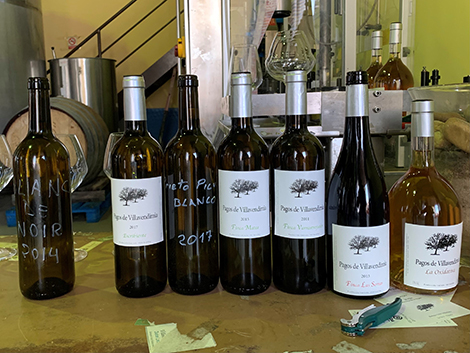The image depicts a selection of wine bottles displayed on a brown surface in a winery setting. There are nine bottles in total, with seven prominently positioned in the foreground and two slightly obscured in the background. Most of the bottles feature the same white label adorned with a black or gray tree design, though the vineyard's name is difficult to discern due to its small print. Notably, one bottle on the right is shorter and wider, labeled "PAGOS" with a silver seal at the top and containing a yellowish-brown liquid. Two bottles in the assortment lack the uniform label and instead have chalk or marker inscriptions, reading "Pinot Blanco 2017" and "Pinot Noir 2014." In the background, there are a few silver tubs and a wooden barrel on its side, along with a yellow wall. A staircase is visible, suggesting an upper level. The scene likely takes place in a French winery, inferred from the style of lettering on the labels and general ambiance.